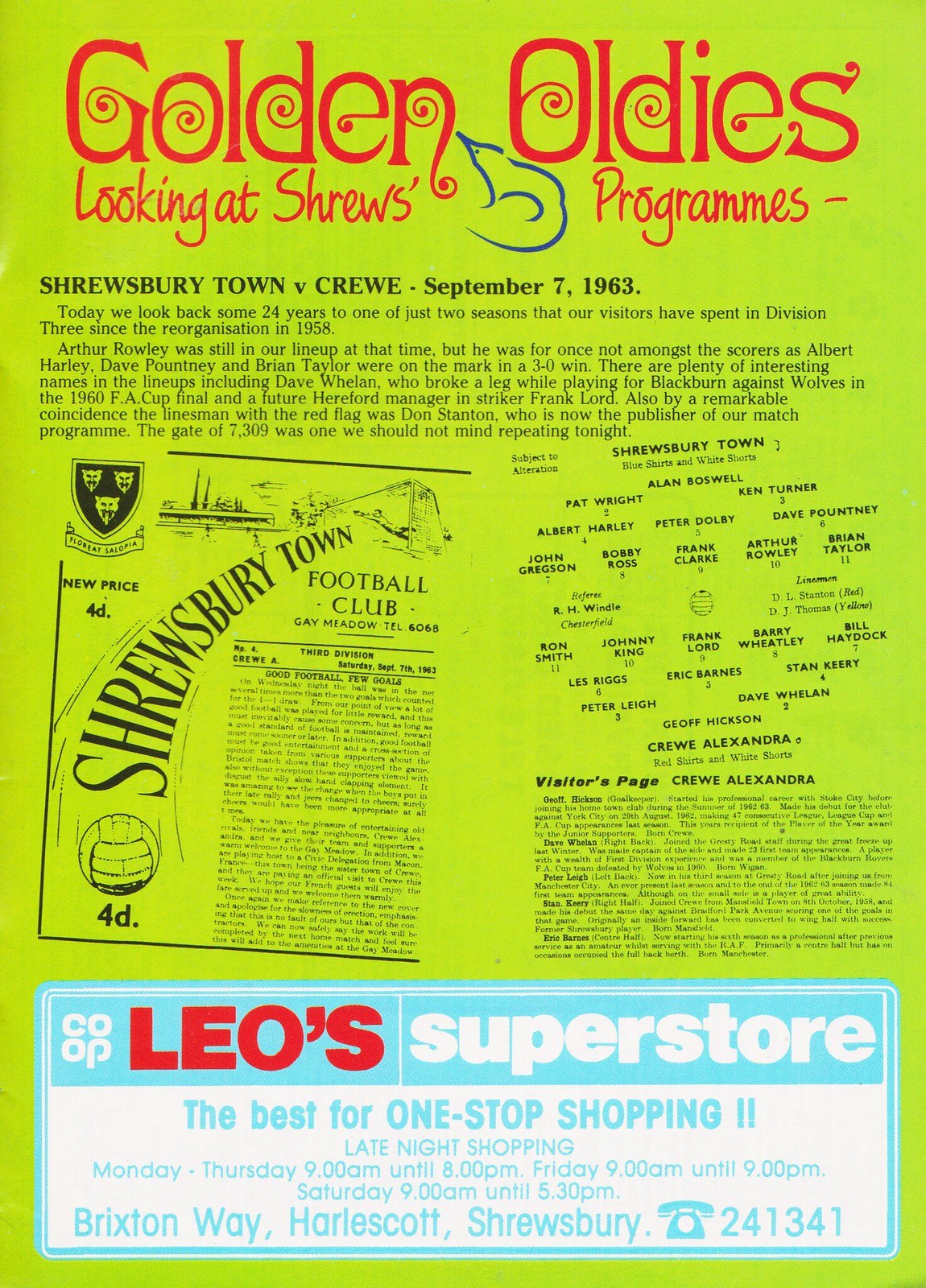The image is of a bright, almost fluorescent green flyer for a football club event. At the very top, in red font, it reads "Golden Oldies," accompanied by a blue outline of a shrew. Beneath this, in black text, it states "Shrewsbury Town v. Crewe, September 7th, 1963," followed by a nostalgic note: "Today we look back some 24 years to one of just two seasons that our visitors have spent in Division III since the reorganization in 1958." This is further elaborated with historical context mentioning players like Arthur Raleigh, who did not score in the game, and highlighting goals by Albert Harley, Dave Putney, and Brian Taylor that led to a 3-0 win. Additionally, it references notable names such as Dave Whelan. 

Further down, the flyer features what appear to be transposed printouts of historical articles or program notes. The one on the left reads "Shrewsbury Town Football Club" with a note about the "New Price, 4D," while the right section simply states "Shrewsbury Town" along with various team names and numbers.

At the bottom of the flyer, an advertisement for "Leo's Superstore" stands out with a white background and blue border. In red and blue text, it promotes "The Best for One Stop Shopping, Late Night Shopping," detailing hours: Monday through Thursday from 9 AM to 8 PM, Friday from 9 AM to 9 PM, and Saturday from 9 AM to 5:30 PM, located at Brixton Way, Harlow Scott, Shrewsbury. The contact number provided is 241341. 

Overall, this vibrant flyer blends nostalgic football history with contemporary advertisements, commemorating a memorable match from 1963.